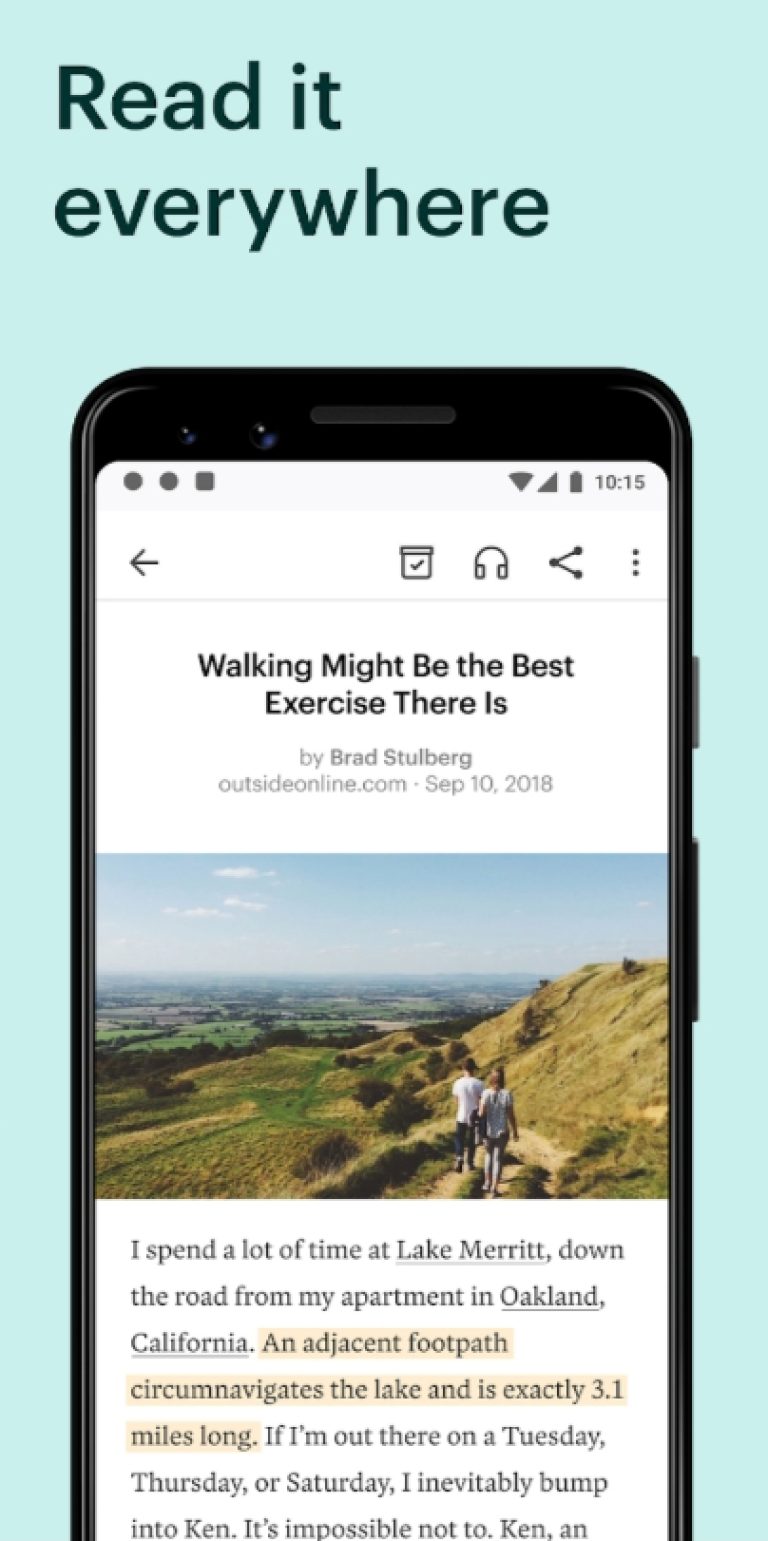This image prominently features a mobile phone displayed on a light turquoise green background. At the top of the image, black text reads, "Read it everywhere." The phone's screen shows various symbols: two gray circles, a gray square, a Wi-Fi symbol, a triangle, a battery icon indicating 10:15, a black left-pointing arrow, a bucket icon with a checkmark, a headphone icon, a less-than symbol with circles on the ends, and three vertical dots representing more options.

Displayed on the phone screen is a news article titled "Walking Might Be the Best Exercise There Is" by Brad Stuhlberg, published on outsideonline.com on September 10, 2018. Below the title, the article features an image of two people, possibly a man and a woman, walking on a trail in a hilly, grassy area with an elevated vantage point. The following text from the article is partially visible and highlighted in yellow: "I spend a lot of time at Lake Merritt down the road from my apartment in Oakland, California. An adjacent footpath circumnavigates the lake and is exactly 3.1 miles long. If I'm out there on a Tuesday, Thursday, or Saturday, I inevitably bump into Ken. It's impossible not to. Ken and..." The text is cut off at this point, leaving the rest incomplete.